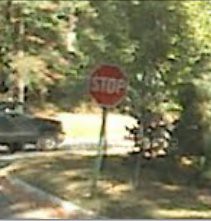This daytime photograph captures a residential neighborhood at the corner of a street, with a slightly bent stop sign at the center, serving as the focal point. The stop sign, mounted on a metal post and surrounded by green grass, prominently features its red octagonal shape with white reflective lettering. To the left, a small black truck, possibly an S10, is visible as it turns at the intersection. The scene is framed by numerous mature trees with lush green foliage in the background, and a hint of a white picket fence. The road gutters are scattered with leaves, suggesting early fall. The image is intentionally blurry, emphasizing the stop sign while other elements, such as the sunlit trees and ground, remain secondary.